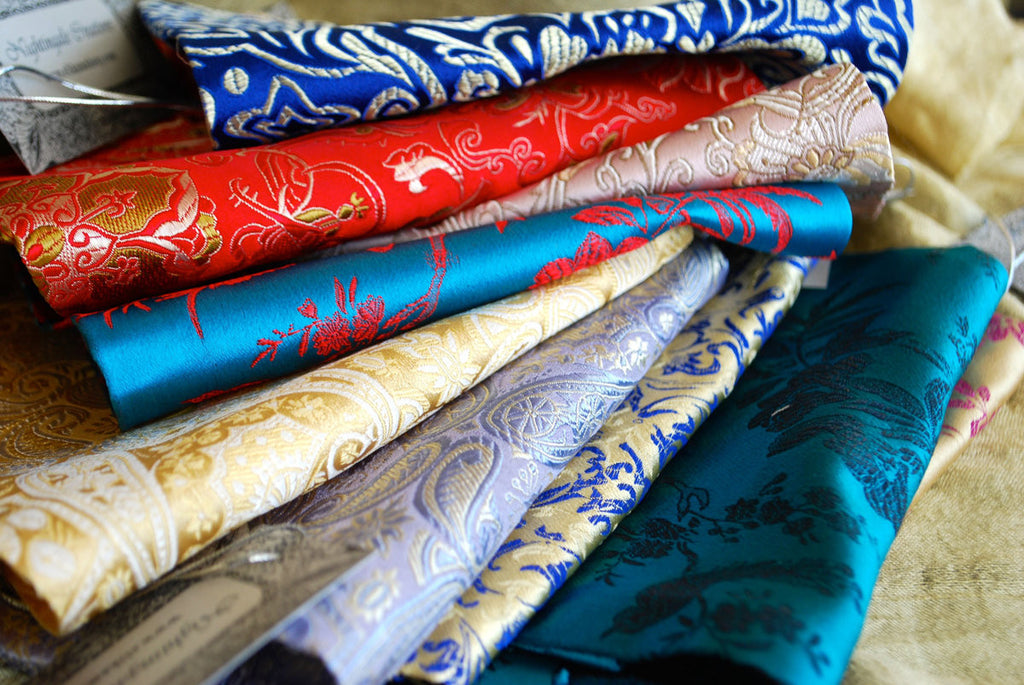This photograph features a meticulously arranged stack of folded, satin-like fabrics, each boasting unique designs and vibrant colors. From the bottom to the top, the first fabric is dark blue with intricate leaf and floral patterns. Above it lies a cream-colored fabric adorned with blue designs, followed by a light blue fabric highlighted with a golden pattern. Proceeding upward, there's a yellow fabric featuring cream-colored designs, eventually leading to a bright turquoise fabric with darker turquoise patterns. Next is another cream-colored piece, showcasing blue patterns, and above it, a striking blue fabric with red detailing. This is followed by a red fabric with gold and silver designs. On top, there's a blue and white fabric, completing the colorful and patterned stack. Many of these fabrics carry embroidered floral patterns, some of which are difficult to discern due to the folds and close stacking of the fabrics.